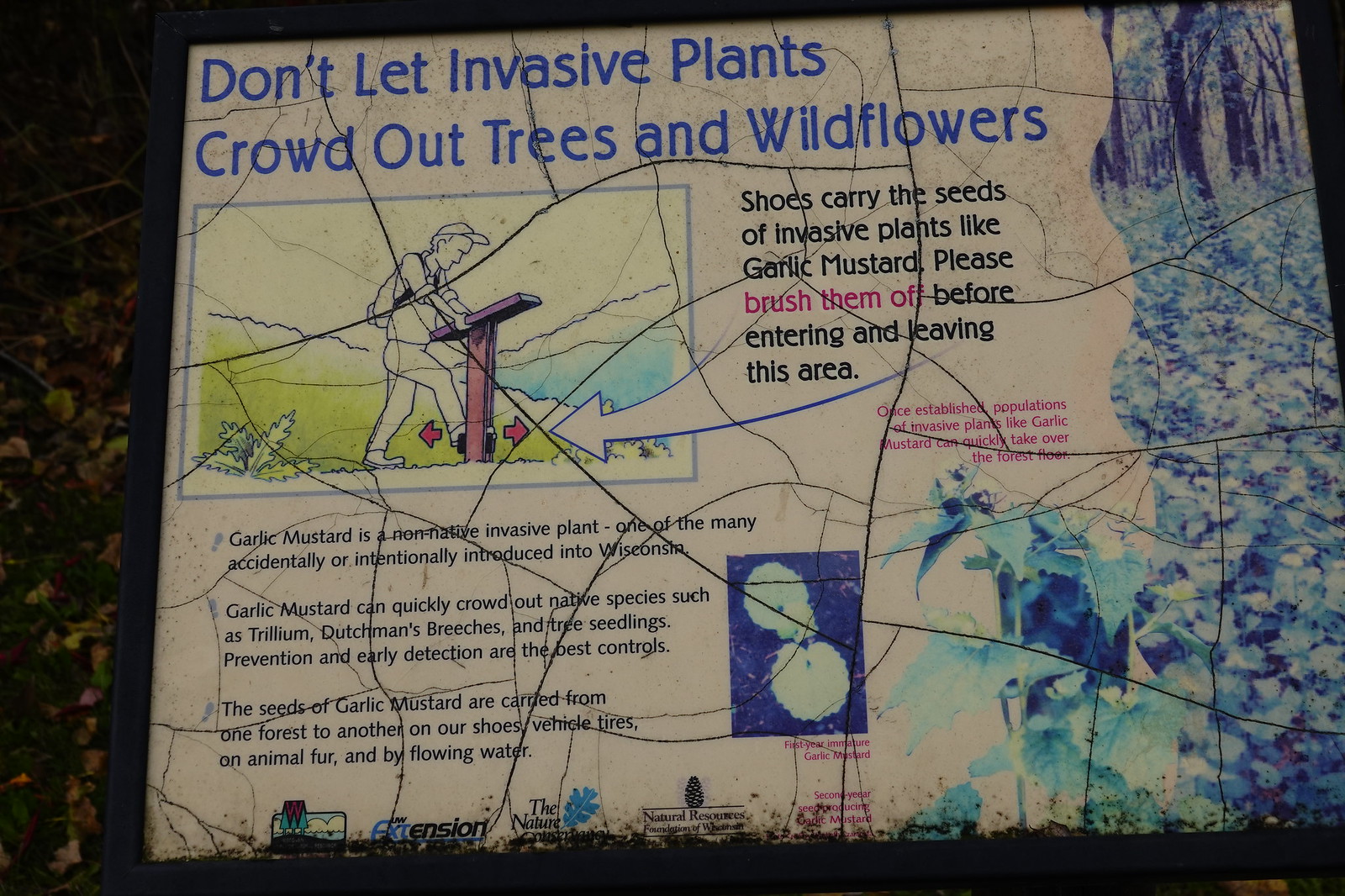The outdoor image captures a weathered and cracked information sign set in a public park, framed by a black metal border. The sign reads at the top in blue lettering, "Don’t let invasive plants crowd out trees and wildflowers." Directly beneath, it continues, "Shoes carry the seeds of invasive plants like garlic mustard. Please brush them off before entering and leaving this area."

On the left side of the sign is a drawing of a man standing outdoors, looking at another wooden sign, with hills and grass in the background. Below the drawing, there are multiple lines of text in black writing, spaced out into distinct groups. The primary text explains, "Garlic mustard is a non-native invasive plant, one of the many accidentally or intentionally introduced into Wisconsin. Garlic mustard can quickly crowd out native species such as trillium, Dutchman's breeches, and tree seedlings. Prevention and early detection are the best controls. The seeds of garlic mustard are carried from one forest to another on our shoes, vehicle tires, animal fur, and by flowing water."

The bottom of the sign features several icons and symbols, five or six in total. To the right of the man’s illustration, there are six lines of text in black, except for three words in pink on the fourth line. On the right edge, there’s an image of trees and grass extending downwards, ending with what appears to be an animal hidden among leaves.

The ground around the sign is covered with leaves in various shades of gray and brown, adding to the autumnal atmosphere. The overall condition of the sign, with its worn and cracked surface, suggests it has endured many seasons of weather exposure.